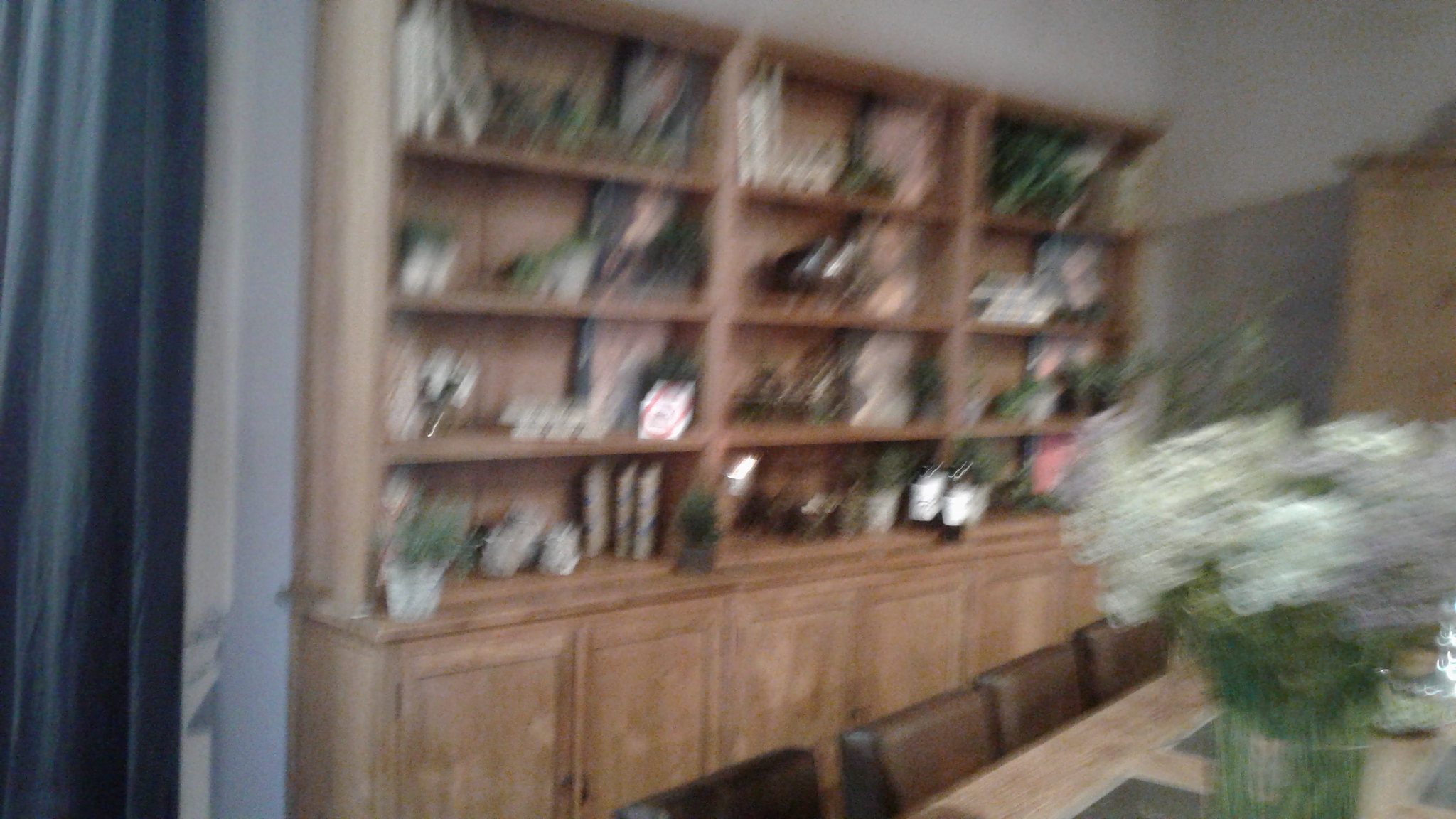This color photograph captures the interior of a room, though it is quite blurry, making it difficult to discern some details. Central to the image is a mid-tone brown wooden dresser, featuring multiple cabinets at its base and four rows of shelves above, each divided into three sections. These shelves display a variety of decorative objects, including what appear to be books, green plants, and bottles with white labels on the bottom shelf. On the left side of the image, a lighter grey door is partially obscured by a blue curtain. To the right, another brown cupboard is visible. In the bottom right corner, a light wooden table is seen, along with four dark chairs pushed in on one side. A vase with tall, round white flowers, likely hydrangeas, stands on the table, accompanied by greyish-green placemats and a small, metallic, shiny object. The wall appears to vary in color due to lighting, ranging from white to light blue. Overall, the room exudes a sense of a dining or meeting area with ample seating and tasteful decor.